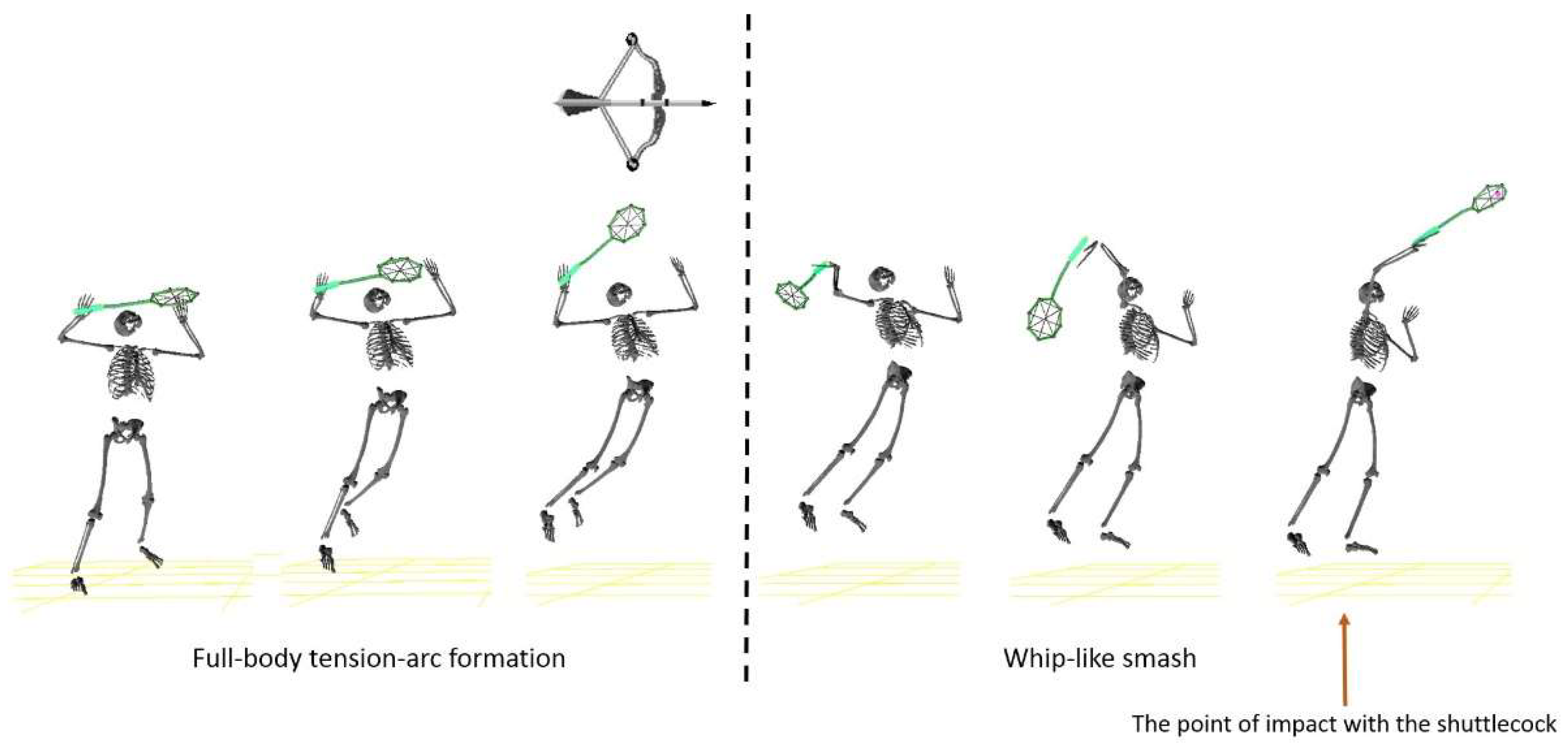The image is a digitally enhanced, horizontally rectangular illustration that depicts six computer-generated human skeletons demonstrating the mechanics of a badminton serve. The background is a plain screen with no additional elements. The illustration is split vertically by a dashed black line, clearly dividing it into two halves.

On the left half, three skeletons are shown in successive positions of the initial stages of serving, with their rackets held overhead progressing to a readiness to strike. Interestingly, over the head of the third skeleton from the left, there is a bow and arrow, adding an unexpected element to the scene. This section is labeled "Full Body Tension Arc Formation" in pale yellow and white text.

The right half illustrates the latter stages, where the skeletons show the follow-through of the serve, culminating in a striking motion labeled "Whiplike Smash." The final figure on this side has a label underneath, specifying "The Point of Impact with the Shuttlecock." The badminton racket in each image is highlighted in green, contrasting against the pale yellow, white, black, and dark brown-red hues of the skeletons and text.

This image meticulously captures the sequential physical dynamics involved in a badminton serve, visualizing both the preparatory and execution phases of the movement.